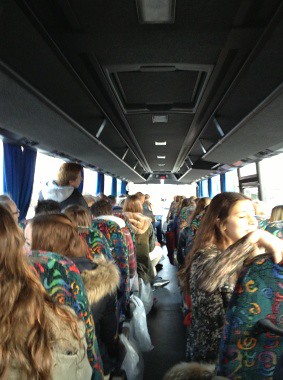In this vibrant and lively photograph of a coach bus interior, we see a crowd of young people, likely high school or college students, seated and engaging with one another. The seats, upholstered in a lively multicolored pattern with swirls, triangles, and squiggles in shades of green, blue, red, orange, and yellow, add an energetic atmosphere. The photograph, taken from the center aisle looking forward, captures the cheerful demeanor of the students, many of whom are girls with long brown hair, clad in winter jackets, some featuring fur-trimmed hoods. The bus is bright and well-lit, with daylight streaming through the large windows flanked by blue curtains. A solitary male with brown hair, standing up in his seat and donning a jacket with a hoodie, looks out the window, adding to the dynamic composition. The gray ceiling with visible air vents completes the detailed interior of this bustling coach bus.